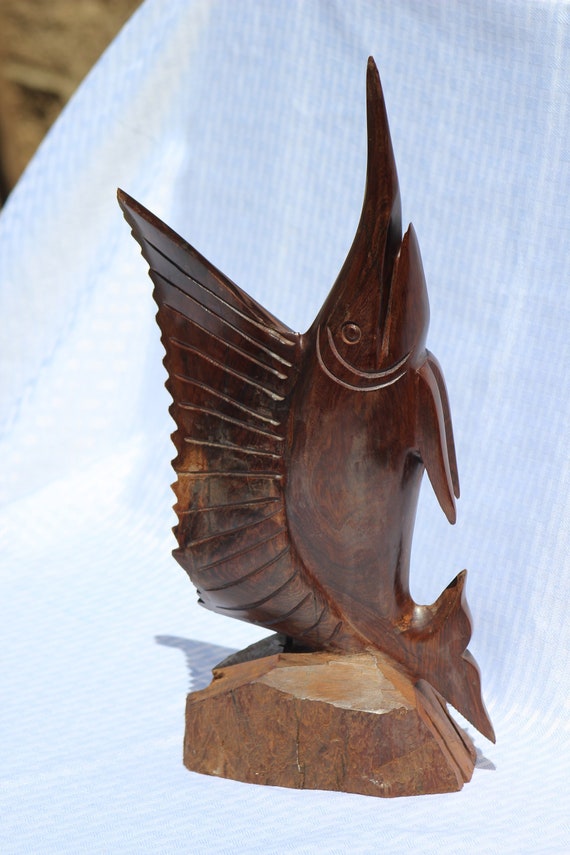This image showcases a meticulously carved wooden marlin sculpture, characterized by its dark brown hue and glossy finish, likely from varnish or shellac. The marlin is perched on a light brown wooden base that rests on a white textured cloth adorned with vertical lines. The marlin's body, sculpted from a single piece of dark wood, features a pointed nose extending straight up with its high dorsal fin also pointing upward, casting a subtle shadow on the light blue background, which resembles a tablecloth. The sculpture captures intricate details, including gills behind the eyes and finely carved fins. The marlin's tail curves downward, its front fins tucked beneath it, and its circular, wide-open eye gives it a lifelike and alert appearance. The upper right-hand corner of the image suggests the edge of a wooden table, adding context to the marlin's display setting.